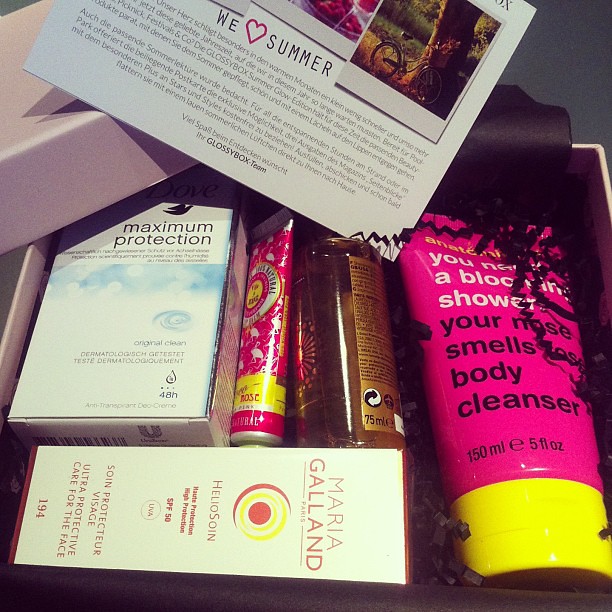The image captures a neatly arranged collection of beauty and skincare products inside a white box adorned with black paper confetti. Dominantly positioned in the center, the box contains an assortment of lotions, cleansers, oils, and creams. Key items include Dove Maximum Protection Original Clean deodorant, a sunscreen labeled Maria Galland Paris Heliosoin HOT Protection SPF 50, and a body cleanser branded with the quirky phrase "You need a bloody shower, your nose smells". Also visible is a small tube labeled with the word "rose", and a clear bottle containing a brown liquid without a visible label. At the top of the box, there's a postcard from the Glossy Box team that reads "We Heart Summer", with additional text in a different language. The photo appears to be taken indoors, possibly in someone’s makeup cabinet. The objects and packaging display a range of colors including dark gray, white, pink, gray, brown, orange, tan, light blue, yellow, and black.